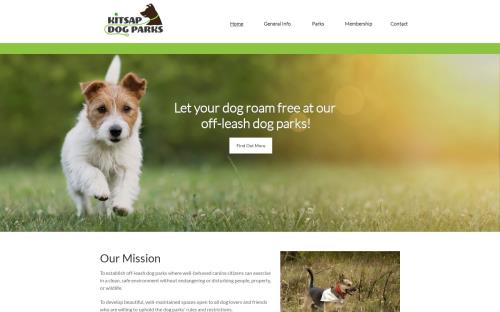**Kitsap Dog Parks Website Overview**

Experience the joy of letting your dog roam free at Kitsap Dog Parks, an off-leash haven for your furry friend. The website features an inviting green banner at the top, showcasing a lively image of a Collie running towards you in a lush, green field. 

Centered on the banner is the welcoming message: "Let your dog roam free at our off-leash dog parks," accompanied by a button below that invites you to learn more. Further down, there's an adorable picture of a Chihuahua, which at first glance looks like a duck, playfully positioned in the park.

Although the mission statement text is small and hard to read, the website clearly focuses on promoting a safe and enjoyable environment for dogs to play without the constraints of a leash. The navigation menu includes links to the Home and Contact pages, among other sections, ensuring easy access to all the necessary information.

Kitsap Dog Parks provide a fantastic opportunity for dog owners to enjoy leash-free areas, making it an ideal spot for well-behaved pets and their owners.